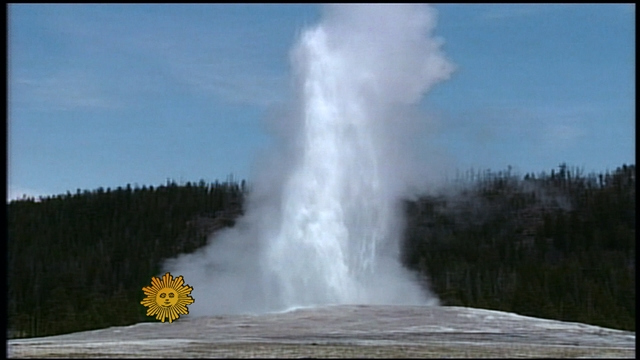The photograph captures a spectacular eruption of the famous Old Faithful geyser in Yellowstone National Park. At the center of the image, a dramatic stream of white water and steam erupts skyward from a rocky, white mount in the foreground. The forceful spray reaches an impressive height, surrounded by various steam clouds and mist, indicating the high temperature of the water. The geyser's eruption forms a striking contrast against the light blue sky, which is dotted with light gray and wispy white clouds, suggesting it is daytime.

The backdrop features a large hill lush with dark green trees, predominantly pine, creating a rich, forested scene. This hillside, running horizontally about halfway up the image, adds depth and natural beauty to the photograph. The land in the foreground is barren, with a grayish, whitewashed appearance, devoid of vegetation, further emphasizing the starkness of the geyser's eruption.

Overlaying the photograph on the lower left side is a yellow sun graphic with a humanoid face and multiple rays emanating from its center. The entire image is encased in a very thin black border, and its photographic realism vividly captures the awe-inspiring natural phenomenon.